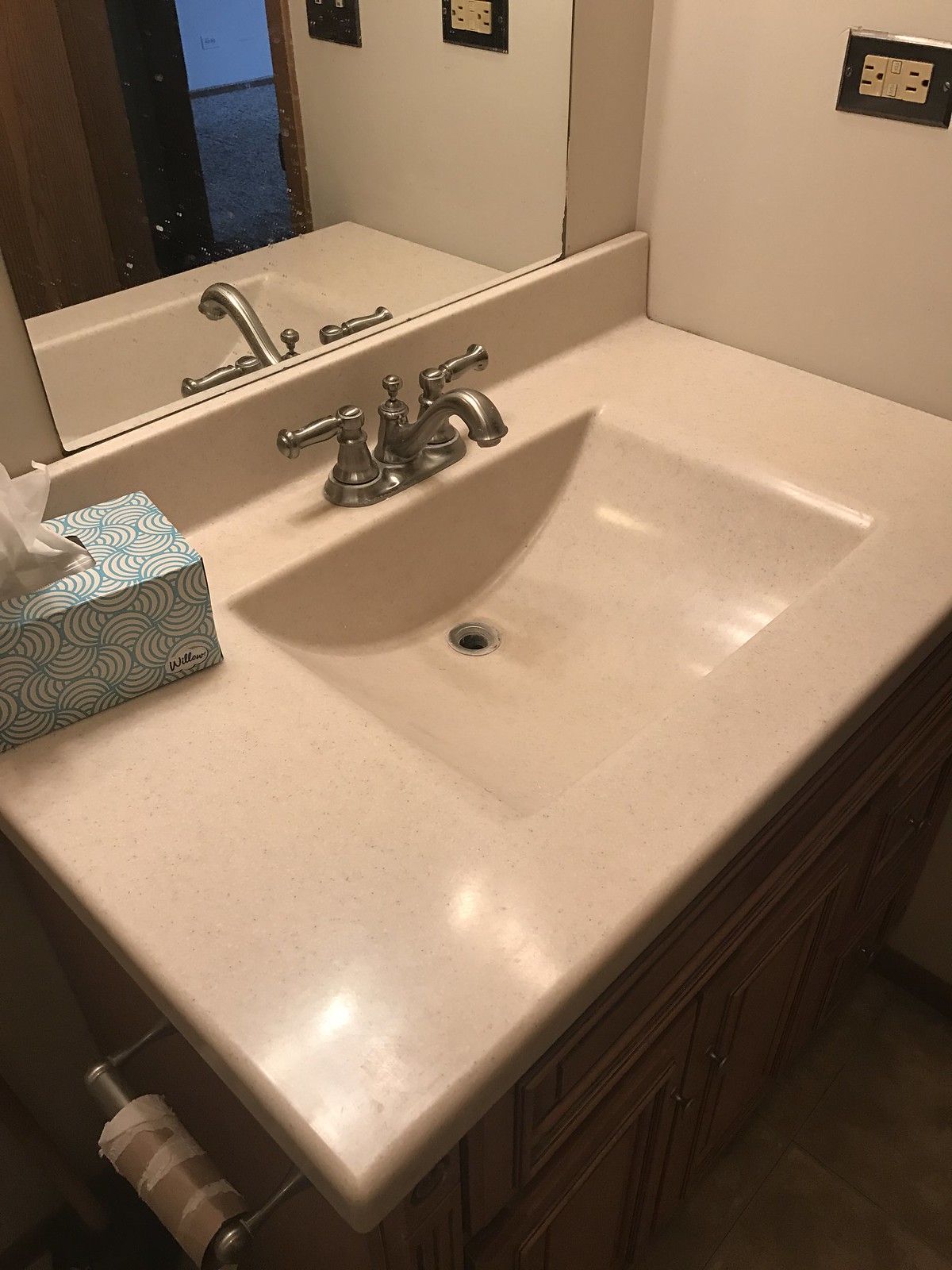This image captures an aging bathroom scene, centered around a modest sink. To the left of the sink, attached to the brown oak cabinetry, is a toilet paper dispenser, holding an entirely empty roll with just a few remnants of white paper clinging to it. The countertop above the cabinetry appears old and worn. The floor is tiled with dated tiles that add to the sense of age in the space. On the wall, there is an older-looking electrical outlet with a metal trim that is installed sideways. 

The smaller mirror above the sink reflects a glimpse into an adjacent room, revealing a space that seems unfurnished, with white walls and brown trim along the baseboard. The room is carpeted in a tan shade, though the hue might appear differently due to the lighting conditions. The light in the bathroom is on, casting a bright glow directly onto the sink area, where all these details come together to form a coherent yet nostalgically aged scene.